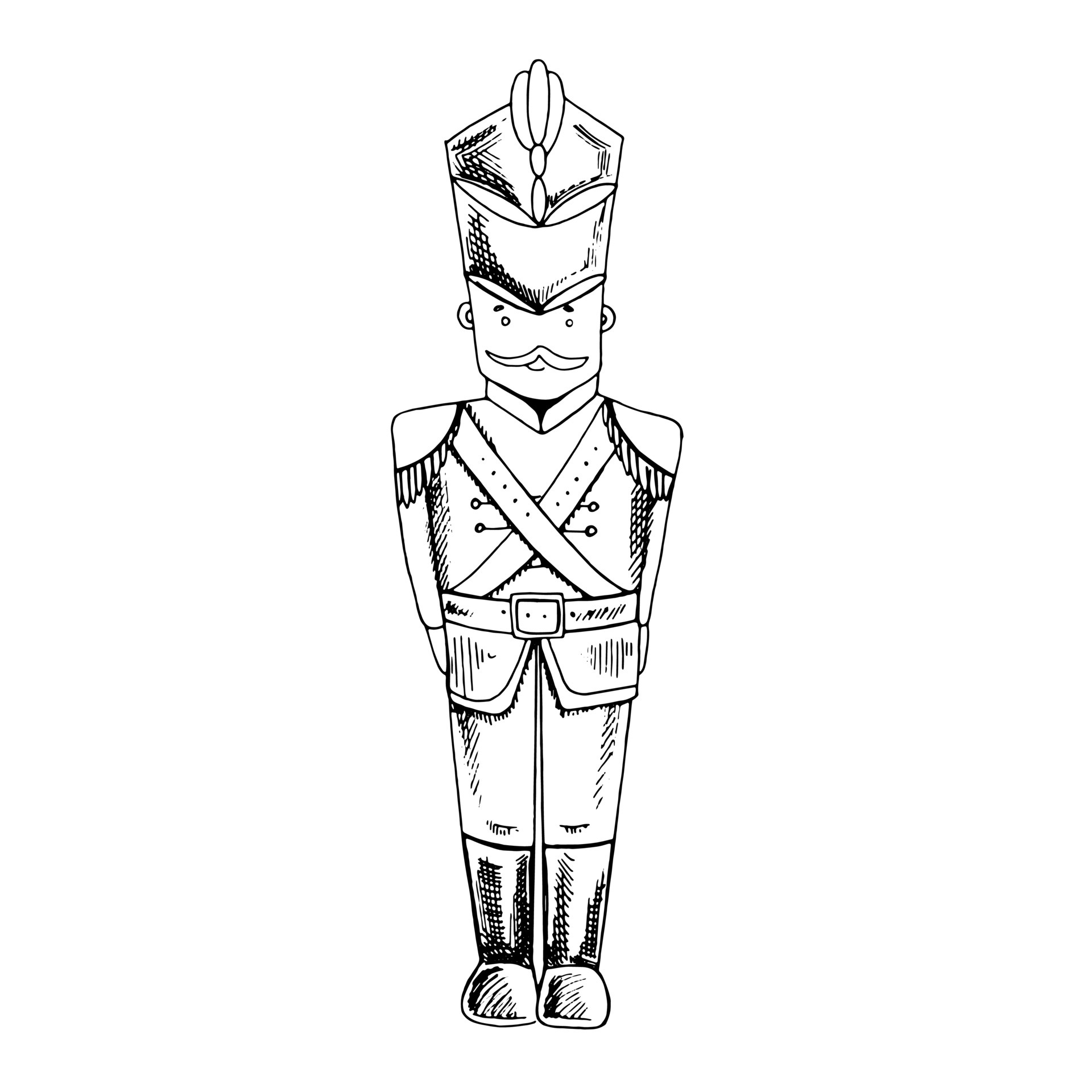The black and white image is a detailed line drawing of a toy soldier standing upright. The soldier is centrally positioned with his arms by his sides and feet together, exuding a stiff and formal posture typical of nutcracker figures. He is clad in a large jacket fastened by a belt at the waist, featuring a distinctive crossed X pattern on the front, shoulder pads adorned with tassels, and secured with a pronounced belt buckle. His pants tuck into large, black boots.

The soldier's face is simplistic, characterized by two small circular eyes spaced apart, darker spots for eyebrows, and complemented by a large, curved mustache. His ears are visible on each side of his head. Topping his appearance is a tall hat adorned with a floral design towards the top portion, with triangular shapes crowning the brim area. The background is plain white, highlighting the black pen or marker sketch, and the overall illustration is clear, showcasing some crosshatch shading to add texture and depth to the drawing.